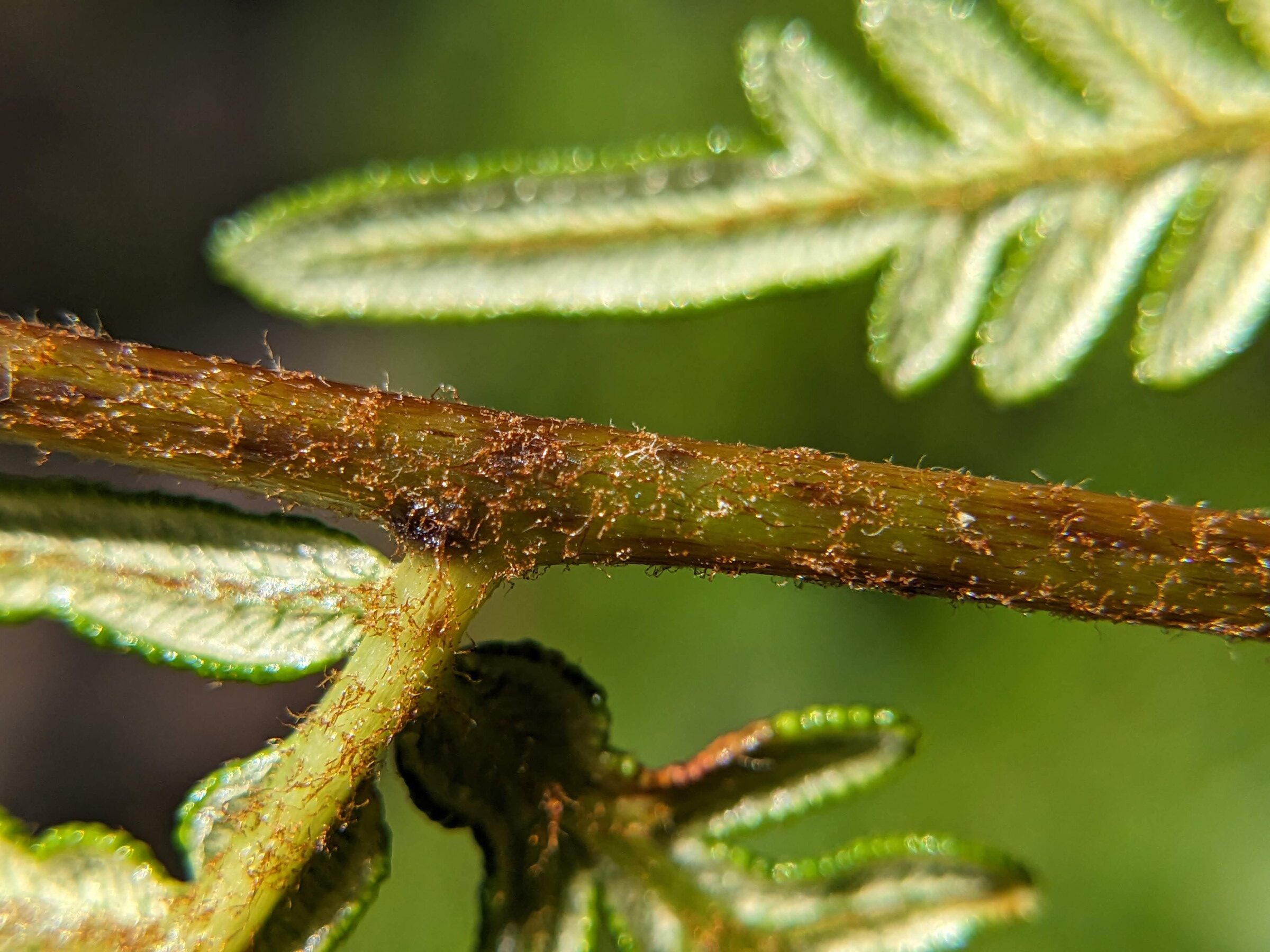This photograph captures an extreme close-up of a textured plant branch or stem, which is the main focus and extends diagonally across the image, forming a T-shape that angles from the center down to the lower left corner. The stem is enveloped in a brownish, fur-like substance that may be natural or possibly a form of microscopic fungus. The primary stem prominently displays a lightish green hue, contrasting with the darker green hue of the main branch. Surrounding this focal area are slightly out-of-focus leaves, some of which appear white on the underside with yellowish veins. These leaves, predominantly pale green edged with darker green minuscule dots, have a unique texture, featuring tiny bubble-like circles around their edges. An elongated leaf, visibly intricate with its almost white underside and distinct veins, stands out near the upper right-hand corner, adding to the intricate detail captured in the verdant, blurred background foliage.